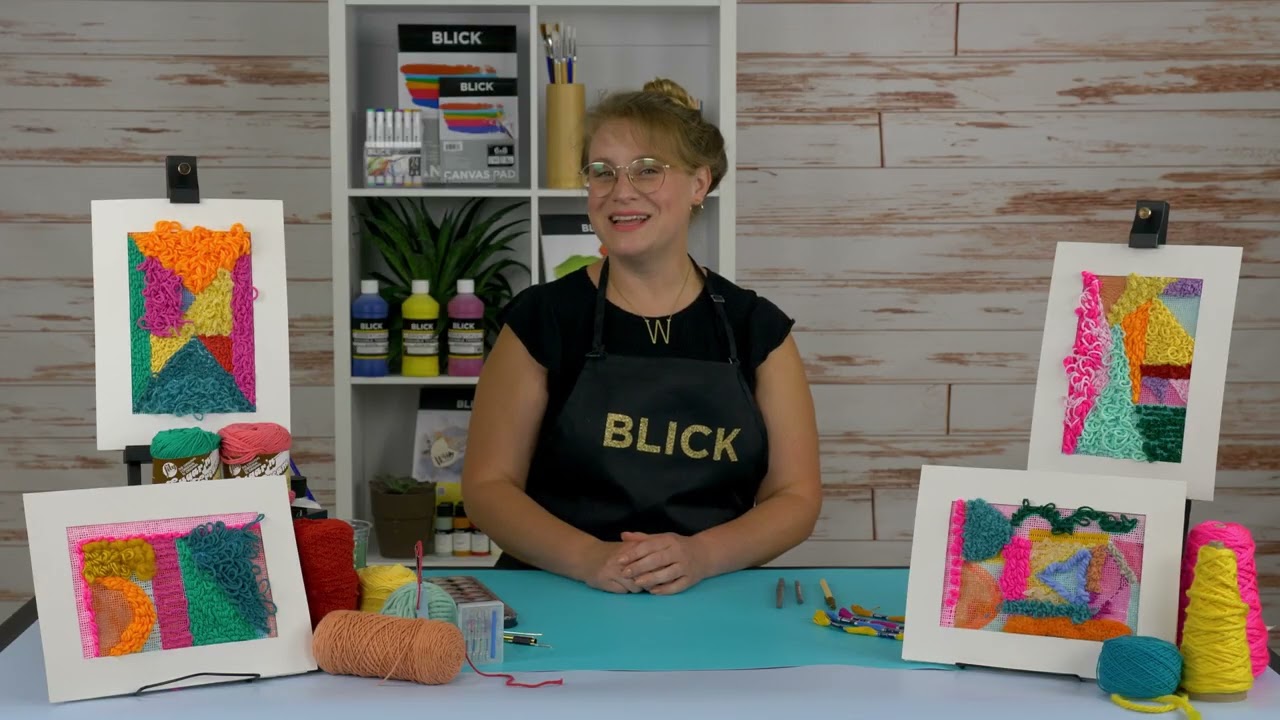A woman, with her light brown hair up and wearing glasses, stands behind a white rectangular countertop adorned with various art supplies. She is centered in the image, smiling, and wearing a black top with a black apron over it that has the word "Blick" in gold letters. Her hands rest on the table in front of her, which showcases a large piece of blue paper, some writing utensils, and several containers of paint in blue, yellow, and pink. Surrounding the paper are different colors of yarn, used to create geometric artwork. Two pieces of this artwork, framed in white, are placed on easels and stands on both the left and right sides of the table. These framed pieces include a mix of colorful designs and possibly some letters. Behind her, the wall appears to be designed with light-colored wood and brown streaks, resembling wallpaper. A white rectangular bookcase filled with additional art supplies is positioned just to her left, providing a backdrop of creativity and organization.